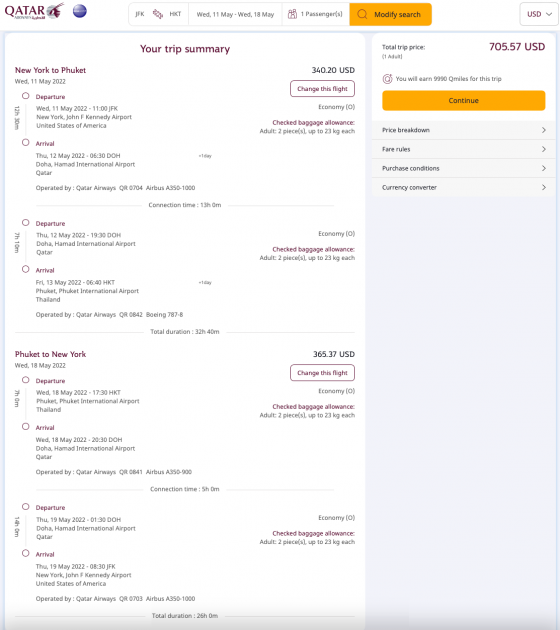The image showcases a detailed travel itinerary for a trip from New York (JFK) to Phuket (HKT) with Qatar Airways. The itinerary is for one passenger traveling from Wednesday, May 11th to Wednesday, May 18th, 2022. 

In the upper left-hand corner, "Qatar" is prominently displayed. The itinerary includes a modification option and displays prices in US dollars, with an orange bar indicating these features.

Key details are:

- **Summary**:
  - Outbound flight: New York to Phuket on Wednesday, May 11th, 2022.
  - Return flight: Phuket to New York on Wednesday, May 18th, 2022.
  
- **Flight Details**:
  - **Outbound Flight**:
    - Departure information
    - Arrival information
    - Total duration: **26 hours 0 minutes**
    - Connection time: **13 hours 0 minutes**
  - **Return Flight**:
    - Departure information
    - Arrival information
    - Total duration: **12 hours 40 minutes**
    - Connection time: **5 hours 0 minutes**

- **Class and Baggage**:
  - Flying Economy class.
  - Checked baggage allowance: Two pieces, up to 23 kilograms each (indicated in purple).

- **Cost**:
  - Total trip price: **$705.57 USD**
  - Miles earned: **$99.90 Q miles**
  - Outbound flight cost: **$340.20 USD** per segment.

Additional options in the itinerary include modifying the search, changing the flight (highlighted in a purple box), checking baggage allowance, and other features such as a price breakdown, fare rules, purchase conditions, and a currency converter. These options are accompanied by arrows pointing to the right. A prominent orange "continue" button is also visible.